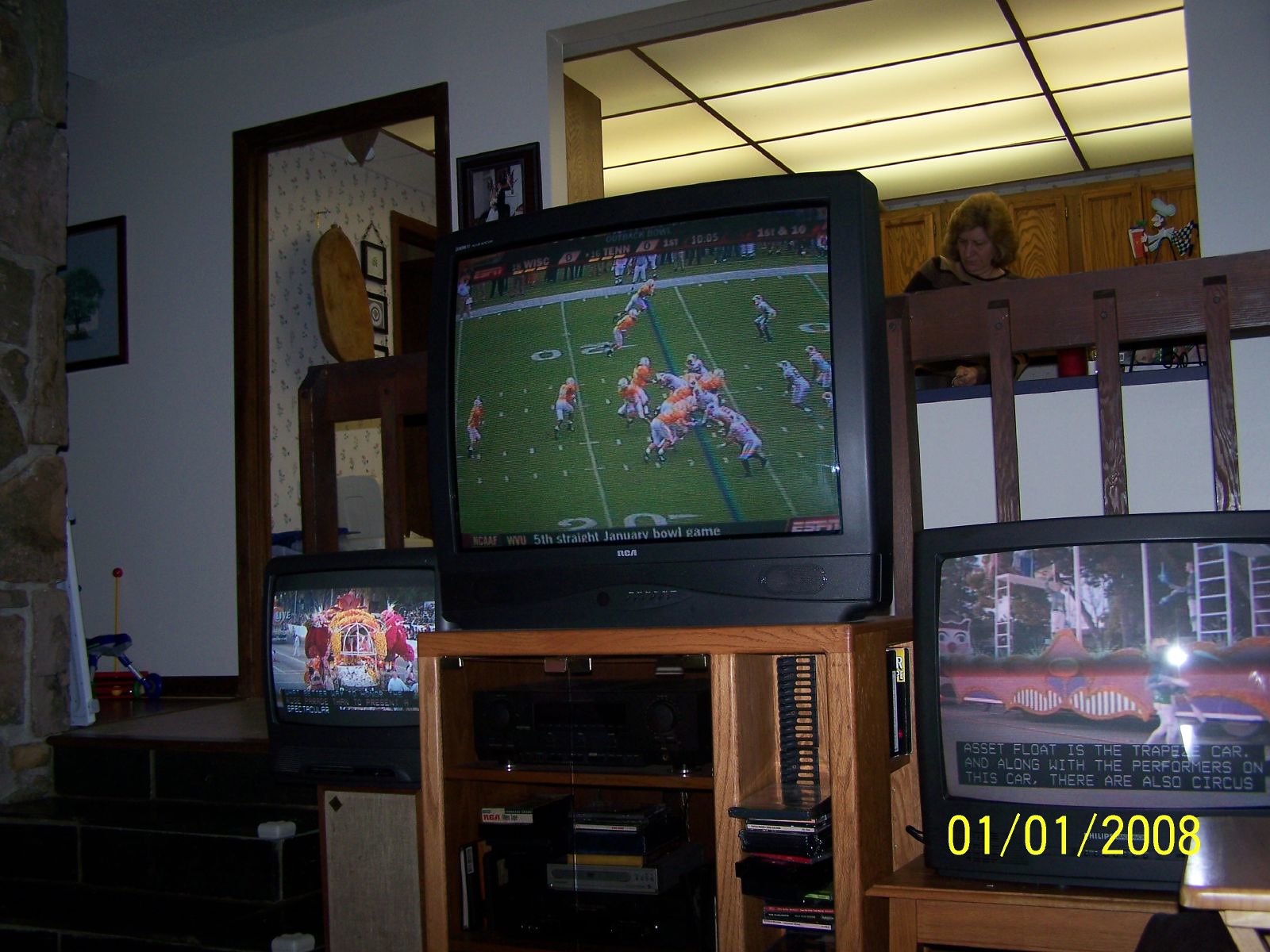This is an image captured in someone's game room or living room, taken on January 1st, 2008, as indicated by the yellow date stamp in the bottom right corner. The room features three old-fashioned CRT TVs arranged side-by-side on wooden cabinets, a setup typical of a sports enthusiast's haven. The largest TV in the center displays a football game with the Denver Broncos, identifiable by their orange jerseys, playing against a team in white. To the right is a medium-sized TV showing what appears to be a parade, specifically mentioning assets related to a trapeze car and circus performers. The smallest TV on the left is airing another event that is not distinctly clear but involves a royal coach.

The setting is warmly detailed with brown wooden cabinetry, a visible stack of DVDs or video game CDs, and additional electronics stored beneath the TVs. In the background, there's a notable cutout in the wall that provides a view into the kitchen area. Here, a woman is seen standing, possibly preparing food, under a drop ceiling with plastic diffusers. The kitchen connects to the living room via a short set of black stairs, which ascend to the elevated kitchen space. The decor includes a mix of black stairs, brown cabinetry, and a noticeable rock wall or fireplace to the left. A kid's toy can be spotted in the hallway, adding a touch of everyday family life to the scene.